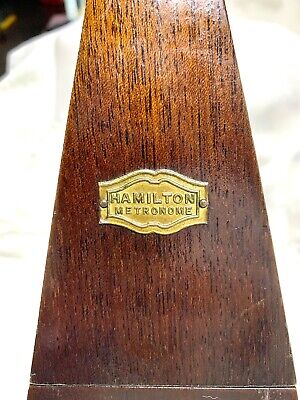The close-up photograph captures the wooden base of a Hamilton metronome, viewed from the backside, focusing primarily on its craftsmanship and details. The piece of wood is triangular and resembles a plank picked from dark, cherry-colored wood, exhibiting prominent dark grains across its surface. It appears highly polished, indicating it has been waxed or coated for a lustrous finish. Centrally fixed to this wooden base is a golden emblem, intricately stamped with the words "Hamilton Metronome," secured with nails or screws. The background is intentionally out of focus, providing a sharp contrast with its bright white hue, thus amplifying the metronome's wooden base as the central element, including the precise interlocking of the planks at the bottom of the photograph.